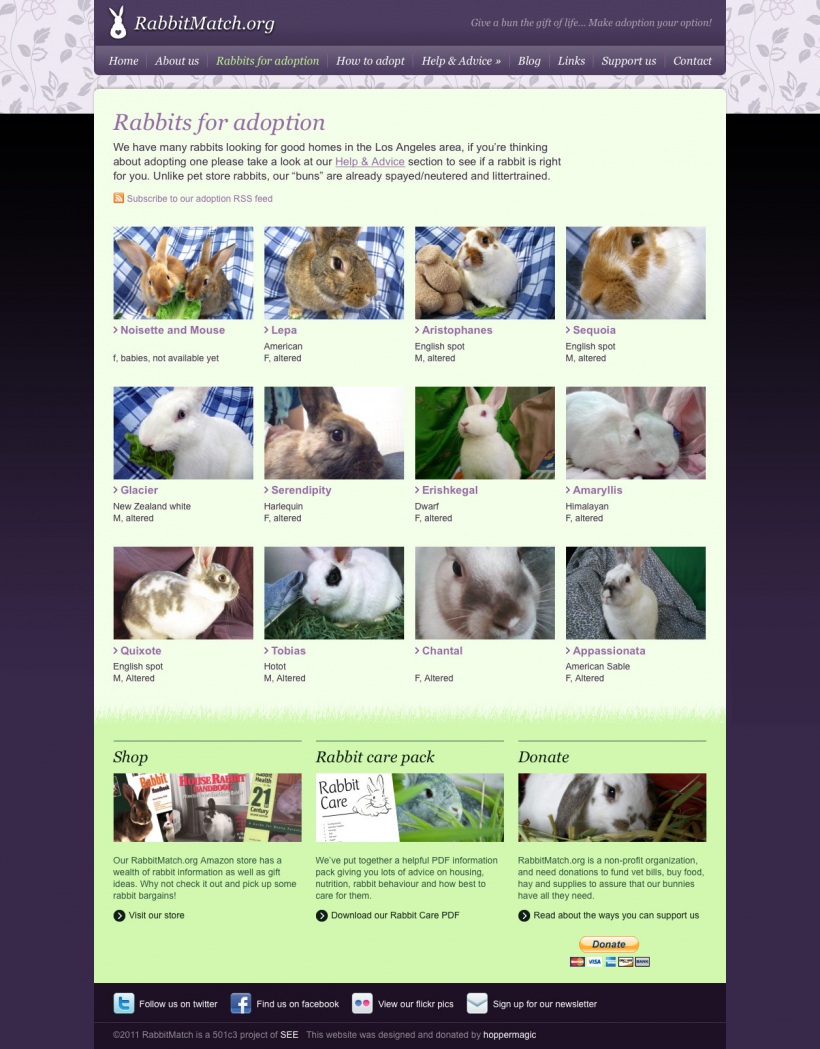Sure! Here’s a cleaned-up and detailed caption for the image:

---

The image is a screenshot from the website rabbitmatch.org. The background features a soft purple hue, complemented by a very light periwinkle top banner adorned with purple leaves or flower stems. Positioned next to the website's name, "rabbitmatch.org," is a cute white bunny icon with a heart-shaped tail. The navigation bar includes options such as Home, About Us, Rabbits for Adoption, How to Adopt, Help and Advice, Blog, Links, Support Us, and Contact.

Below the banner, in small text, it reads: "Rabbits for Adoption. We have many rabbits looking for good homes in the Los Angeles area. If you're thinking about adopting one, please take a look at our Help and Advice section to see if a rabbit is right for you."

The page displays several pictures of rabbits available for adoption. The first picture shows two rabbits: one brown and the other blonde. The caption appears to mention something about "Mouse," but it's unclear. The second picture features a single brown rabbit, possibly named Lopa, though the text is very small. Following this are images of:

- A white rabbit with brown markings
- Another white rabbit with brown markings
- A white rabbit
- A gray rabbit
- Several more white rabbits
- A white and gray rabbit
- A white rabbit with black marks around its eyes
- A white rabbit with a dusty-colored face
- A white rabbit with black on its nose